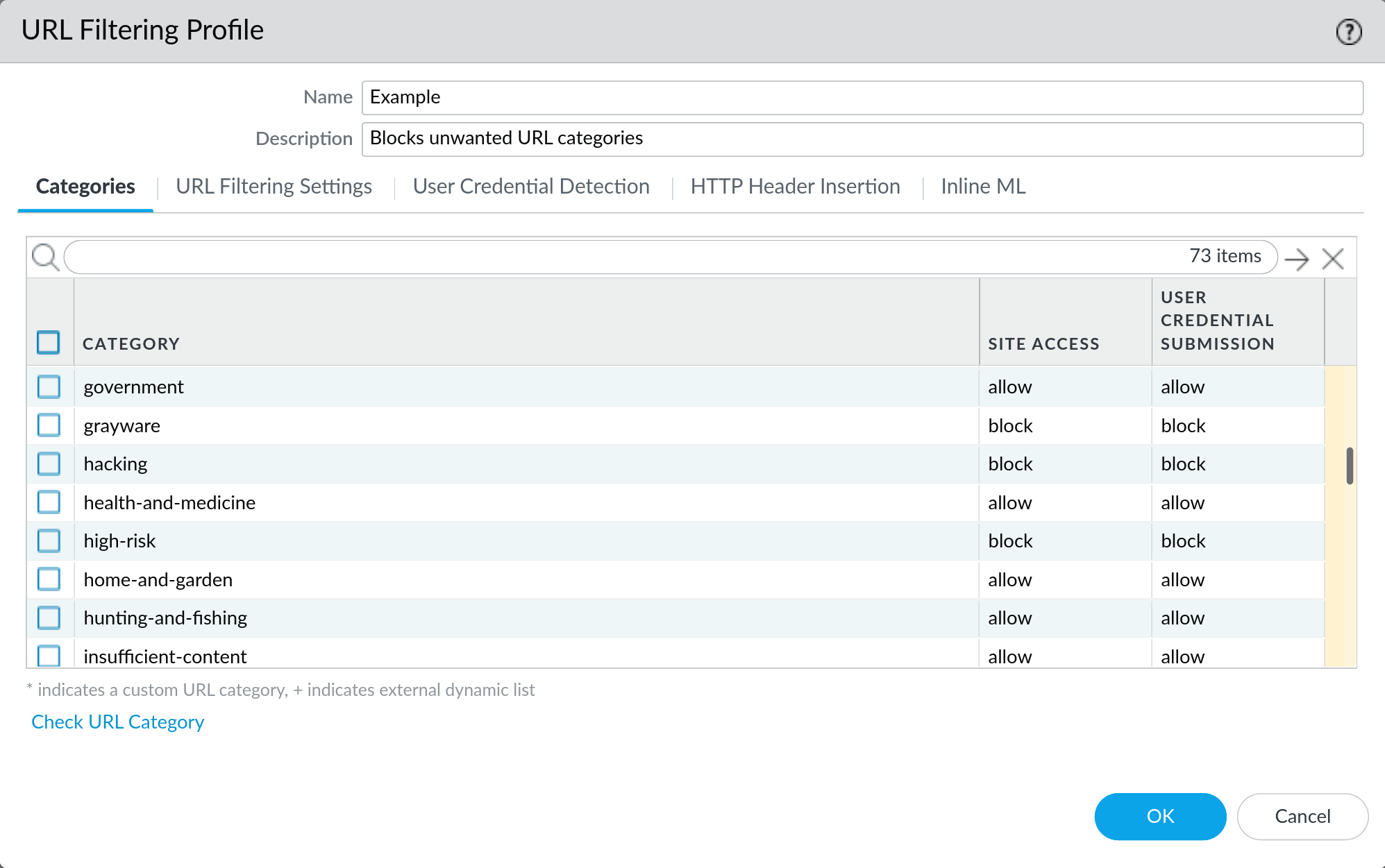The image depicts a detailed screenshot of a URL filtering profile configuration settings on a website. At the top, the webpage title reads "URL Filtering Profile," indicating that the user is managing settings to control access to various internet categories. There is a name field labeled "Example" and a description field that reads "Blocks unwanted URL categories."

The main content of the page displays multiple tabs: Categories, URL Filtering Settings, User Credential Detection, HTTP Header Insertion, and Inline ML. The "Categories" tab is prominently selected, underlined in blue, and displayed in bold.

Within the Categories tab, there is a list of URL categories with associated tick boxes for each category. The listed categories include Government, Grayware, Hacking, Health and Medicine, High Risk, Home and Garden, Hunting and Fishing, and Insufficient Content. None of the tick boxes are selected.

To the right of the categories list, there is a column titled "Site Access," designating whether each category is allowed or blocked. According to this column, the access settings are as follows:
- Allowed: Government, Health and Medicine, Home and Garden, Hunting and Fishing, Insufficient Content
- Blocked: Grayware, Hacking, High Risk

Further to the right, there is another column titled "User Credential Submission," which mirrors the same allow/block configuration as the "Site Access" column.

This detailed configuration page exemplifies a meticulous and organized approach to managing user access and submissions to different online content categories.